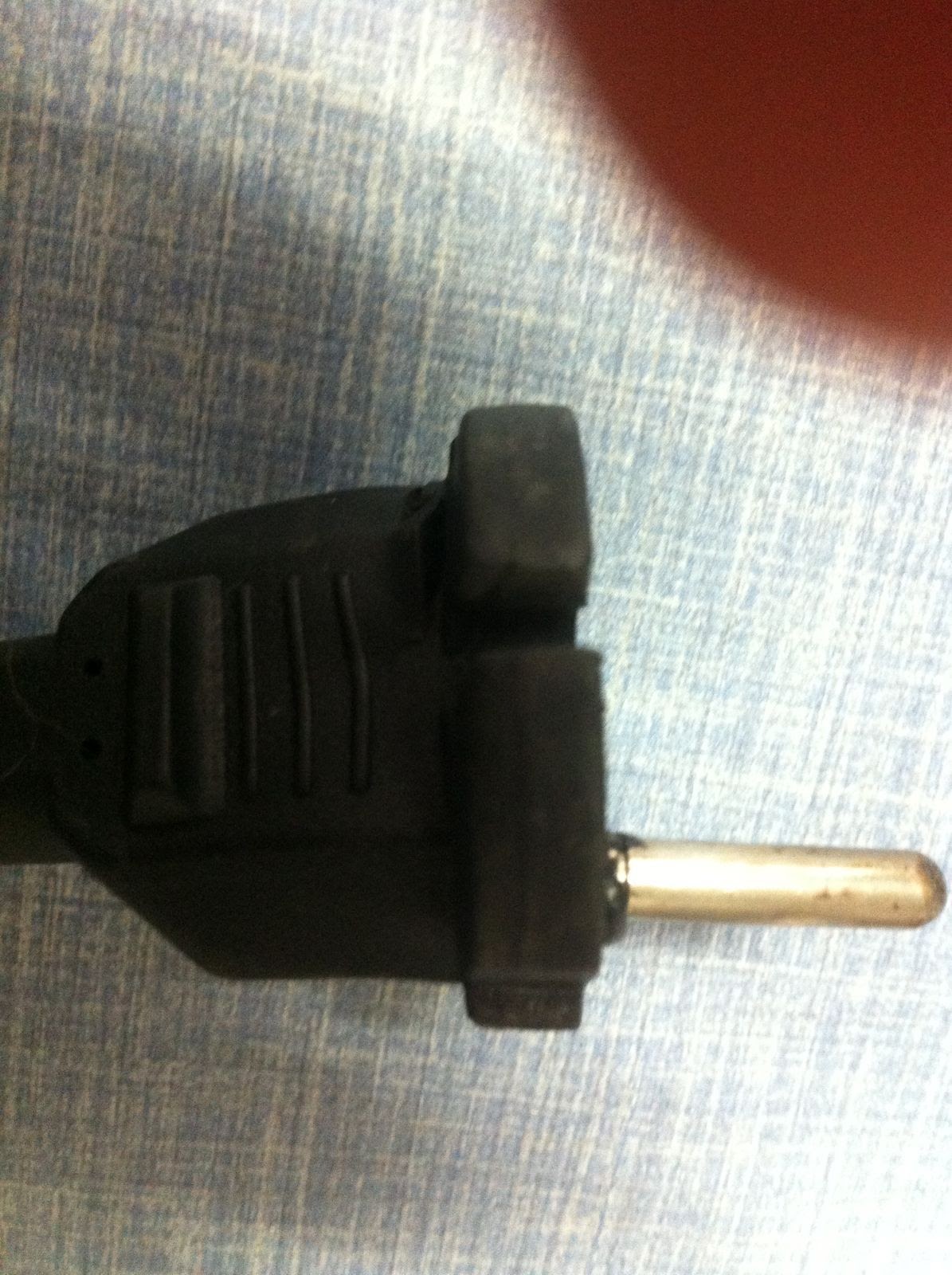The photograph is a close-up image of a black electrical plug made from a rubbery material, placed upon a blue and white woven fabric background, potentially denim or a similar textile. Notably, the plug features a single cylindrical grounding prong, gold in color, with the two flat conducting prongs missing or broken off, giving it a worn, rugged appearance. The focus of the image is centered on the broken plug, with the grounding prong prominently displayed. In the upper right-hand corner, the blurred presence of a person's finger suggests an accidental inclusion while taking the picture. The image is backlit from the top, casting light onto the bottom portion of the plug.